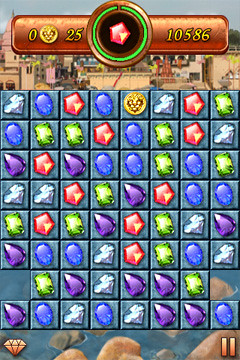The image depicts a colorful video game screen, likely from a smartphone. Dominating the screen are various vividly colored jewels, including red star-shaped gems, green rectangular gems, and oval-shaped blue sapphires. Near the bottom of the screen, there is a diamond-shaped icon in a pale golden yellow color, followed by two vertical golden marks. At the top of the screen, there's a status bar displaying a zero on the left side and the number 25 in the center, with a green-rimmed dial highlighting the red star gem. The current score, prominently visible, is 10,586 points.